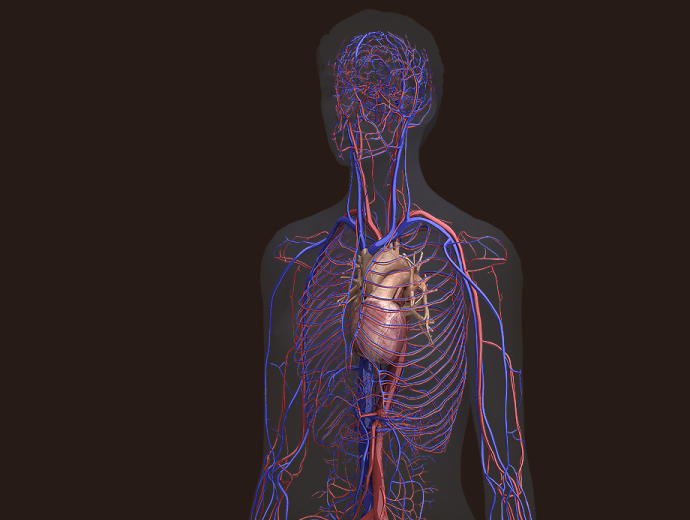The image presents a detailed 3D medical diagram of the human circulatory system, showcasing the intricate network of veins and arteries within a transparent male silhouette on a black background. The semi-transparent figure reveals the entire upper body, including the rib cage, heart, and major blood vessels extending from the head, through the neck, down both arms, and branching out through the chest into the stomach area. The veins are depicted in blue, while the arteries are in red, creating a vivid contrast. The heart is shown in tan with a distinct red lower section. The veins and arteries vary in thickness, with some appearing thick and round, while others are small and thin, emphasizing the complexity of the circulatory pathways.